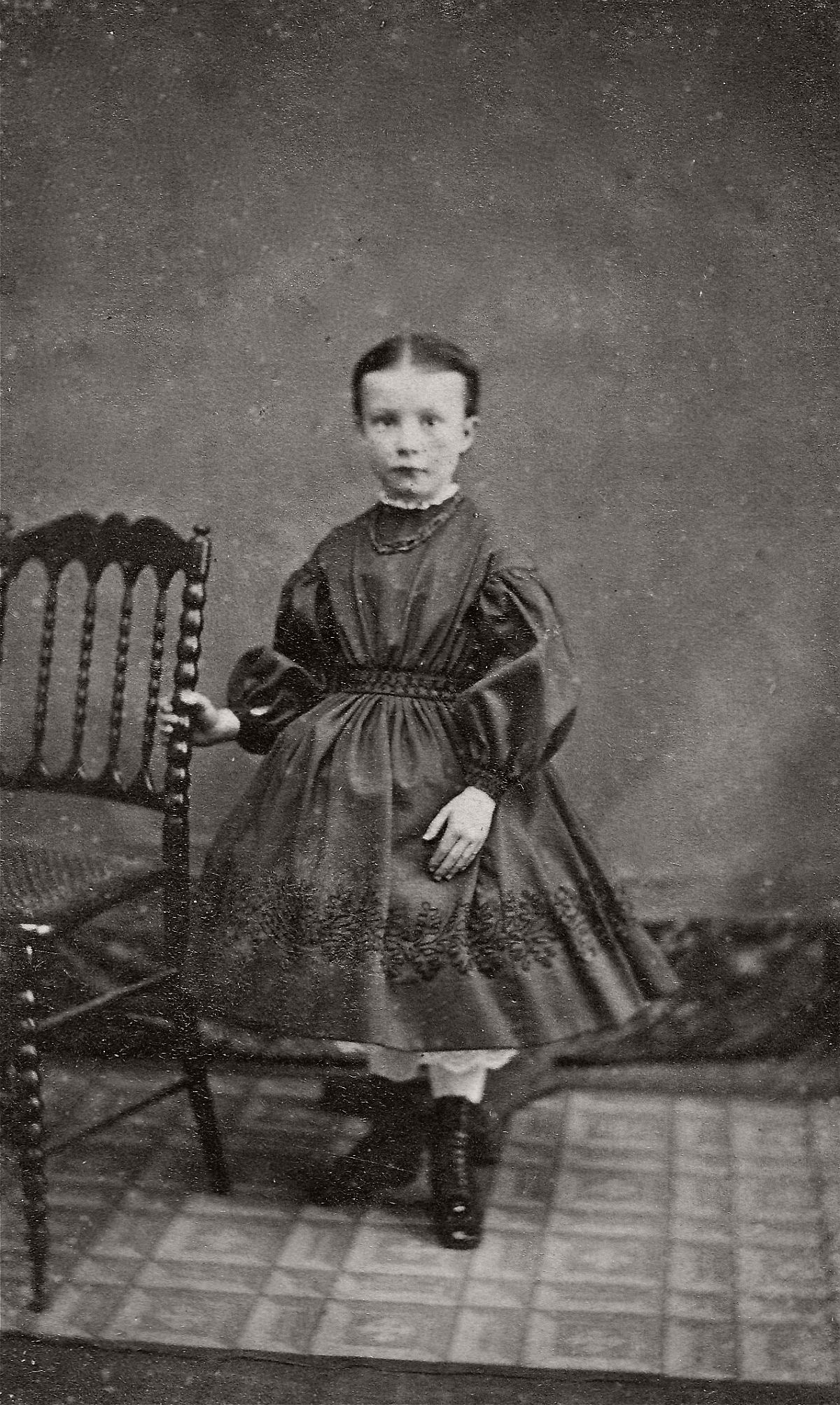In the photograph, a young girl, likely around six or seven years old, stands centered in the frame, gazing solemnly at the camera. The image is a black and white portrait, giving it an antique feel, possibly from the late 1800s. She is dressed in a dark, fluffy dress that flares out at the bottom, resembling a ballroom gown, and has intricate embroidery near the hem. The dress has ruffled fabric at the wrists and is cinched at the waist with a waistband or belt.

Her short hair is parted in the middle and combed to the sides, creating a neat and formal look for the era. A white choker adorns her neck, adding to the outfit's ornate detail. She wears shiny, high-laced black boots over what appears to be white tights or undergarments that peek below the dress.

The little girl’s right hand grasps a small wooden chair to her side (left in the picture), which partially extends out of the frame. Her left foot is slightly ahead of her right, suggesting a poised stance. Behind her, the backdrop consists of a gray wall with a darker baseboard, indicating an indoor setting. She stands on a square, plaid-patterned rug, which covers a dark floor.

Her expression is serious, typical of photographic portraits from that time period, capturing the solemnity and formality expected in such historical images.